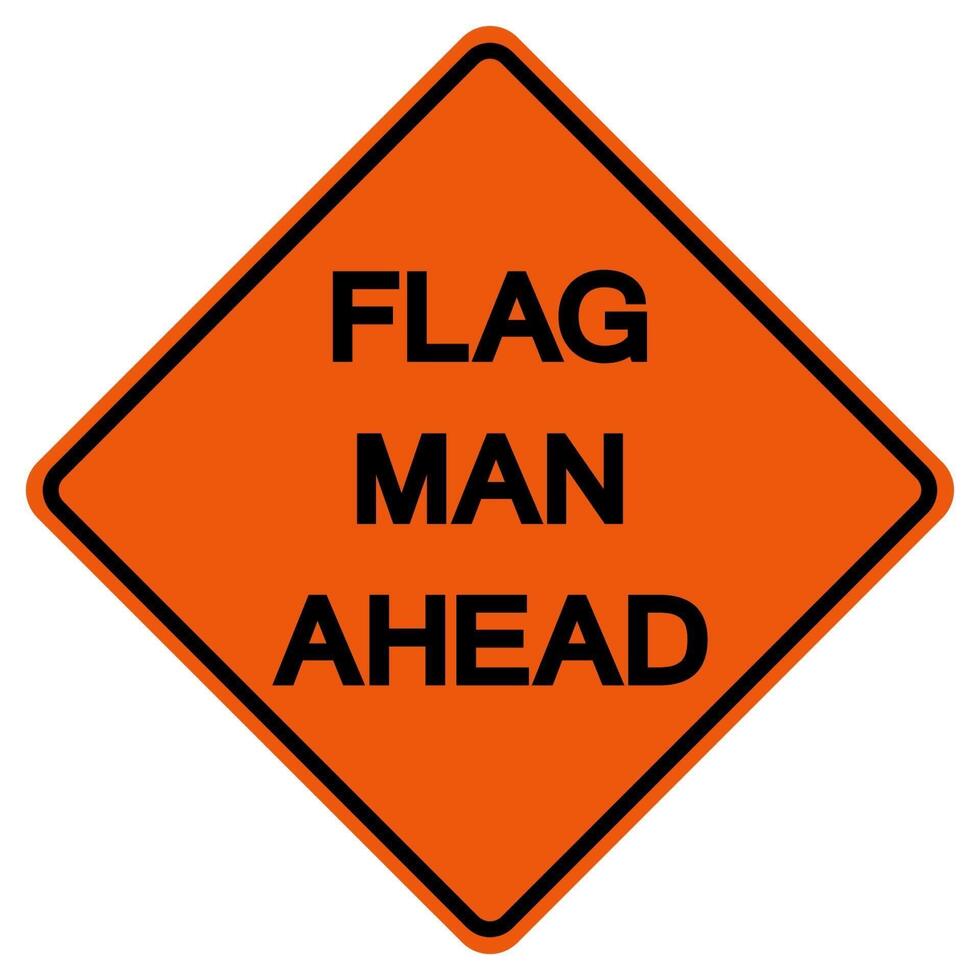This image features a prominent diamond-shaped construction sign against a white background. The sign, which appears square but is rotated so that one corner points upward, is a bright, attention-grabbing orange. Encircled by a black band that adds sharpness and clarity, the sign stands out vividly. In bold, black, and simple uppercase font, the sign reads "FLAG MAN AHEAD." The lettering spans almost edge-to-edge, optimizing the sign's visibility and ensuring it effectively warns drivers to slow down. The stark contrast between the black text and the bright orange background enhances readability, making the sign easy to notice and understand even at a distance.